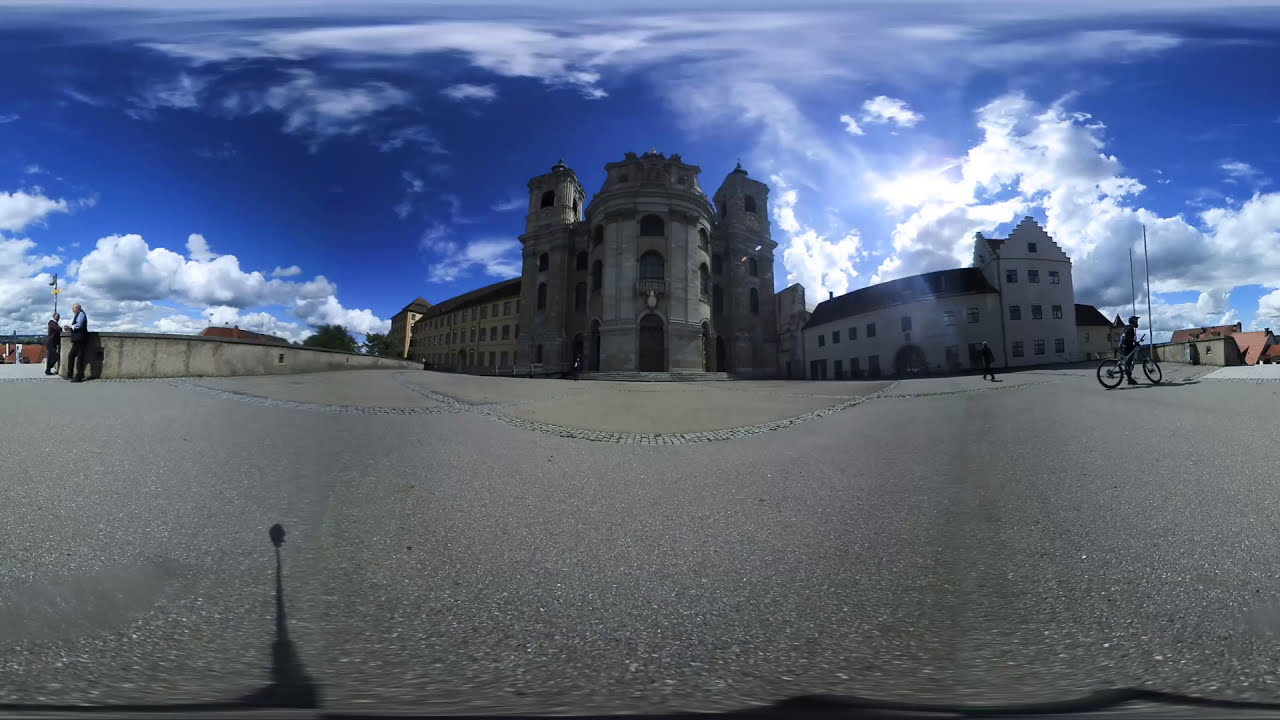The image depicts an old, potentially several-hundred-years-old castle or cathedral located in what appears to be a European city, possibly Romania. The structure, which dominates the center of the image, rises about three to four stories high, with prominent towers flanking both the left and right sides. The photograph is taken from a low angle, making the building seem even more imposing and grand. In the midground, there is a barrier extending from the main building, where two people are standing. To the right of the scene, there's a slightly newer and shorter building featuring a Dutch-style stepped gable, enhancing the European architectural ambiance. The setting seems to be a town square, as inferred from the open, spacious area that is largely empty save for a few individuals, including a bicyclist and two older people. The tranquil atmosphere is complemented by a mostly blue sky dotted with intermittent clouds, through which sunlight filters, casting a bright light over the scene. The overall impression is one of historical grandeur set against a peaceful, almost vacant urban backdrop.